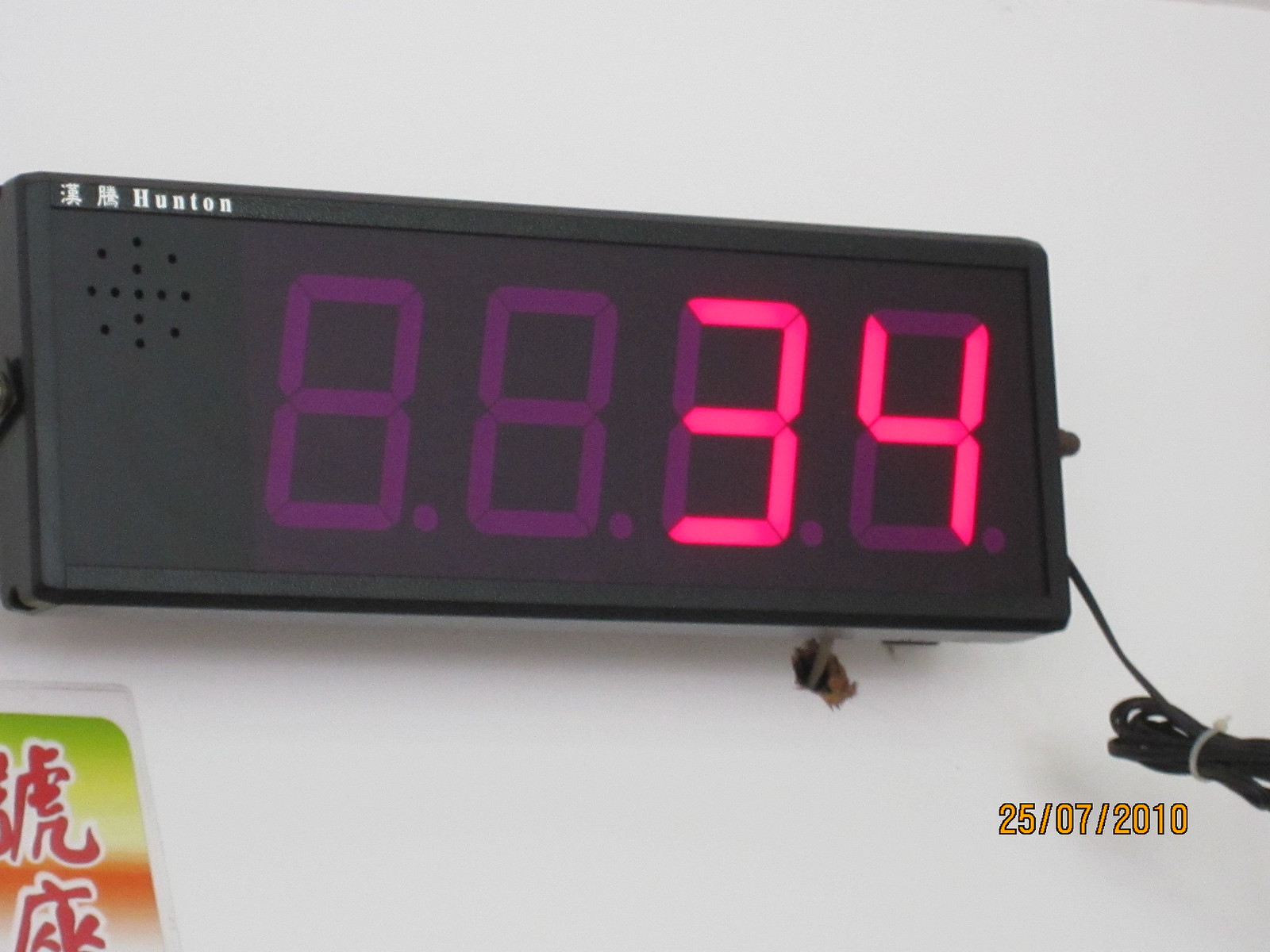This image features a black plastic digital clock or timer mounted on a white wall. The clock's LCD screen prominently displays pink numbers "34" against a black background, with faint placeholder digits "8.8." visible in a muted hue. Above the numbers, there are the words "Hunton" and some Chinese characters, likely denoting the brand or model of the clock. A cord extends from the bottom right corner of the clock, trailing out of the frame. The photograph is timestamped with the date "25/07/2010" in a yellow font with a black border, situated in the bottom right corner. In the bottom left corner, partially visible, is an item featuring Chinese characters in bright colors, seemingly on a golden sticker-like material. This minor element hints at the context, though it remains partly obscured. The overall simplicity of the photograph suggests it might have been taken casually rather than for professional purposes.